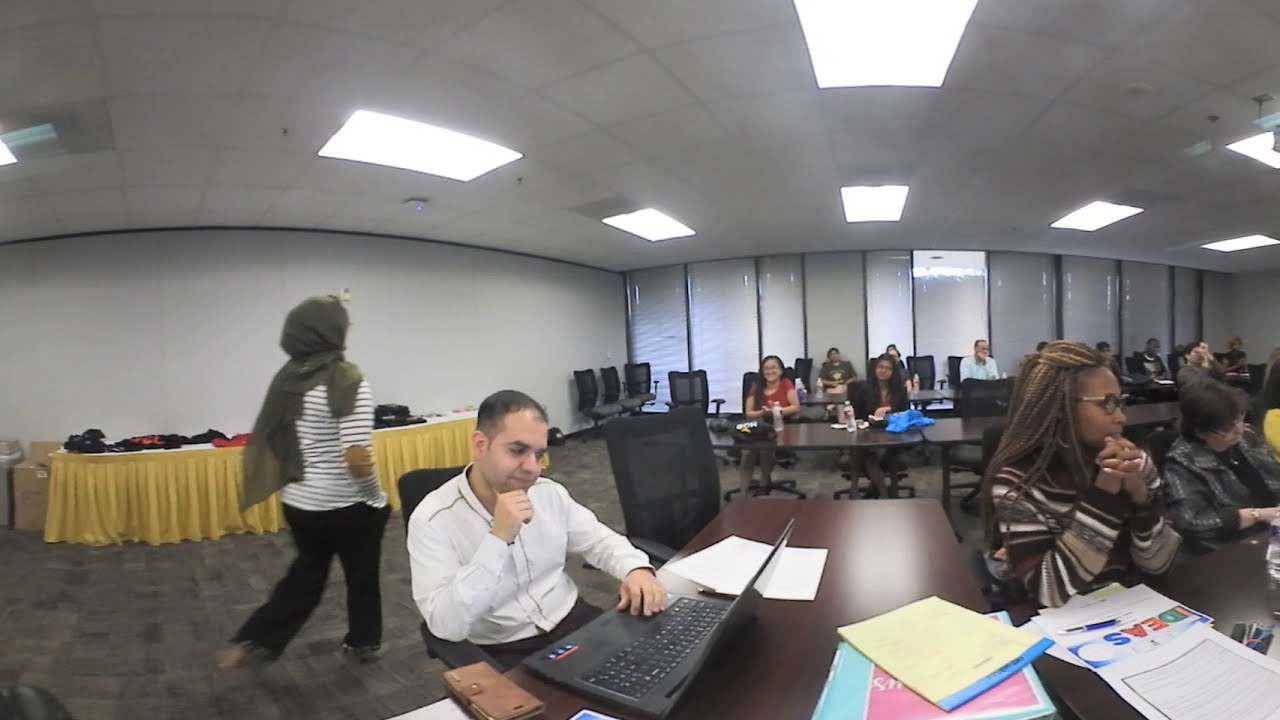The grainy, low-resolution image appears to be a screenshot from surveillance footage capturing a large, bustling office conference room filled with people. The room features white ceiling panels with square lights, and long windows with closed blinds along the back wall. The primary subject of the image is a man of mixed heritage, seated at a brown table near the center. He is dressed in a white button-down shirt with black trousers and is engrossed in reading something on his laptop. His hand rests on his chin contemplatively, with his laptop open in front of him and a brown leather-cased phone to its right. Papers are scattered across his desk.

On the left side of the image, a large table with a yellow curtain draped across it can be seen, appearing to hold various items. The back wall, another focal feature, is white and lined with tall windows. 

In the foreground, to the right, there is a woman with braided hair and glasses, wearing a striped jumper in shades of brown and white, alongside a woman in a green headscarf. She walks across the room wearing a black and white t-shirt and black trousers. Both women are seated at tables, engrossed in their own activities.

The room appears to be setup for a major business meeting or professional class, with people dressed in smart attire, seated on black office chairs, and various paperwork spread across the tables, indicating a busy and professional atmosphere.